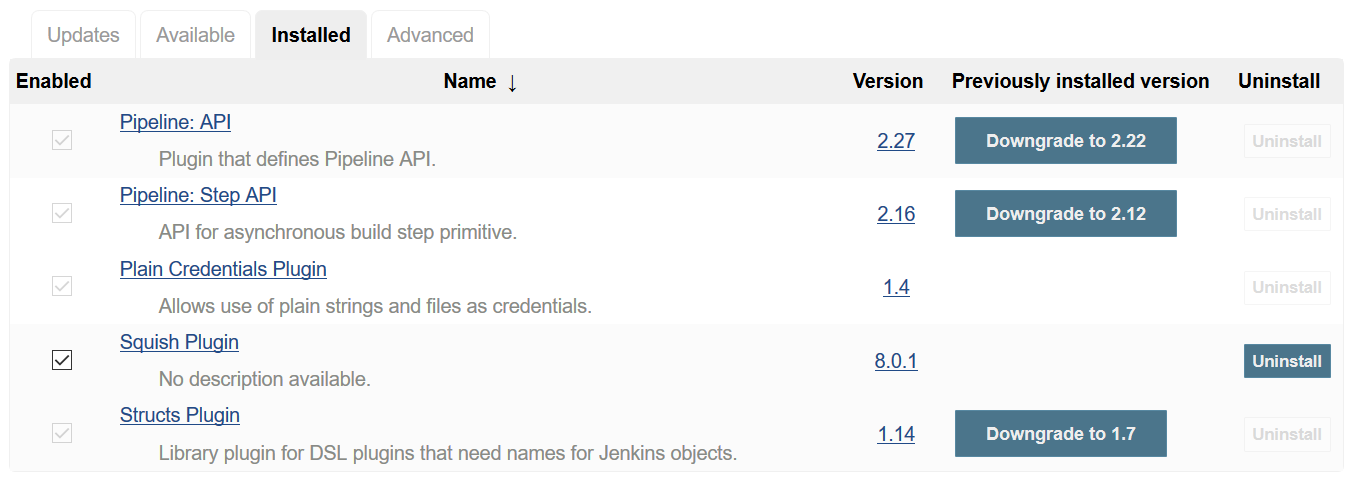The image displays a software update interface with multiple checkboxes indicating available plugins for installation, uninstallation, or update. There are five distinct rows, each representing a different plugin. Each row includes the plugin name, the current version, a previously installed version, and options for enabling or uninstalling the plugin.

1. **Pipeline API Plugin**: This plugin defines the pipeline API and step API, and supports asynchronous build steps. Current version: 2.27, downgraded to 2.22.
2. **Plain Credentials Plugin**: Allows the use of plain strings along with credentials. Current version: 2.16, downgraded to 2.12.
3. **Squish Plugin**: No description available. Current version: 1.4, downgraded to 1.7.
4. **Strux Plugin**: A library plugin for DSTL (Defence Science and Technology Laboratory). Current version: 8.0.1.
5. **Library Plugin**: A generic library plugin. Current version: 1.14.

Each plugin is accompanied by checkboxes for managing its installation status—whether to update or uninstall it. The interface features blue rectangles, possibly highlighting actions or attention areas. There are also visible notes on the downgrade versions, indicating a rollback from the previously installed versions. The design and organized layout suggest a user-friendly interface for managing plugin updates and configurations.